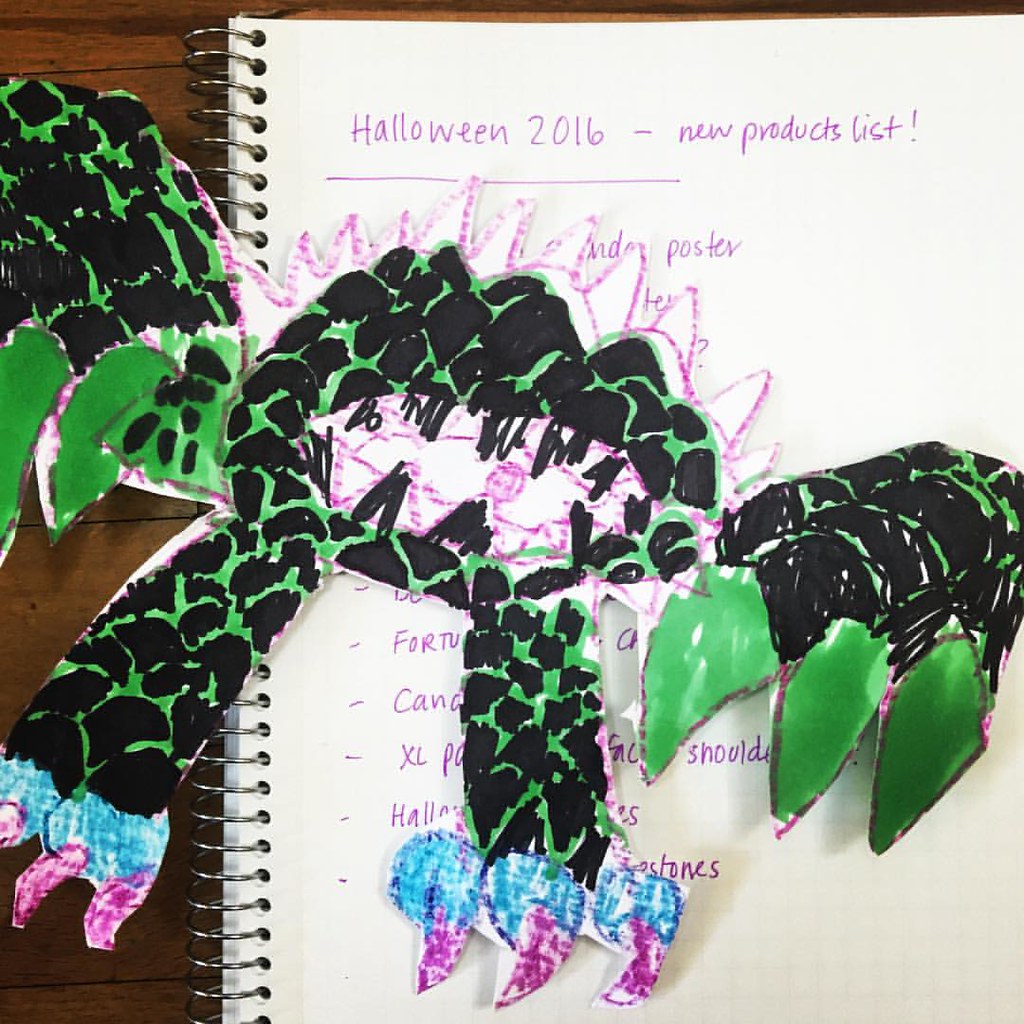The photograph, presented in a square format, captures a white spiral-bound, unlined notebook lying open on a wooden table. The page is headed with the handwritten title in purple marker: "Halloween 2016 - New Products List!" Below the title, a list of items is present, though the text is obscured. Angled across the notebook is a vibrant cutout, seemingly crafted from construction paper and hand-colored with crayons and markers, depicting a fantastical creature resembling a dragon or monster. The creature features black scales on a green body, prominent green claws, and blue feet with purple talons. Its mouth, wide open and toothy, intriguingly displays a pink eyeball. White spikes with pink outlines run along its back. The home-made, childlike aesthetic of the monster figure adds a playful contrast to the otherwise straightforward setting of the notebook, emphasizing the thematic focus on Halloween.